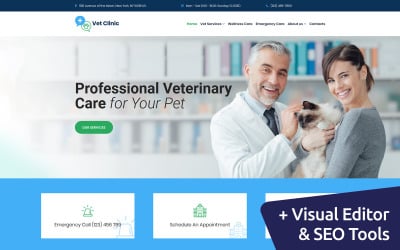The screenshot features a layout of a webpage, starting with a black horizontal header at the top, which contains barely legible blue writing. Below the header, the background is predominantly white. On the left side, there's a logo, subtly indented about a quarter of the way into the frame. To the right of the logo, in bold black text, the words "Vet Clinic" are displayed. Towards the far right, miniature menu options are visible.

Below this section, a central rectangular image depicts a male veterinarian on the right and a woman on the left, with a pet situated between them. To the left of this picture, bold black text reads "Professional Veterinary Care," followed by the phrase "for your pet" in regular black text. Underneath this text, a green oval button with white lettering is present.

At the bottom of the image is an aqua blue rectangular section containing three squares, each with an icon or logo and a line of black text beneath. The rightmost square is partially obscured by a dark blue square extending from the lower right corner. Inside this dark blue square, white text features a plus sign followed by the words "Visual Editor." Below that, an ampersand symbol is followed by "SEO Tools."